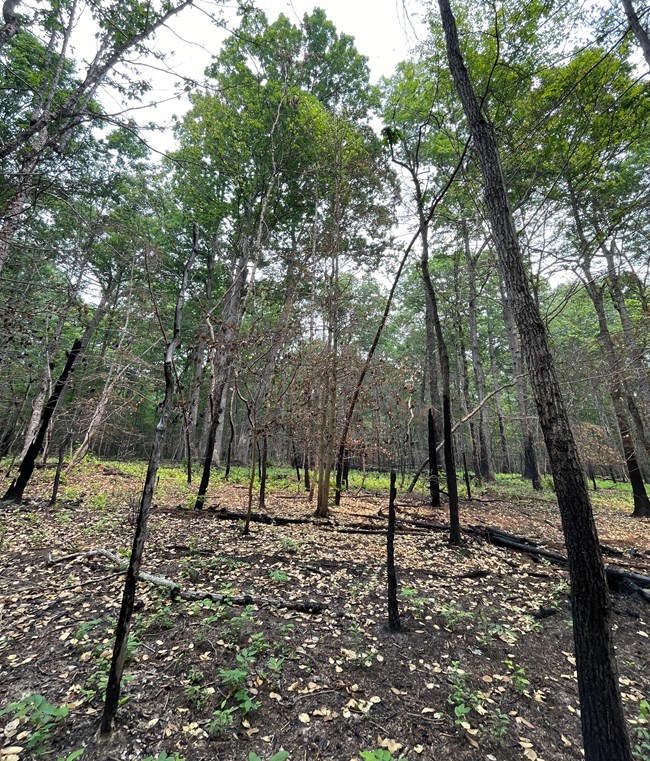The image captures a serene forest scene with a slight incline, viewed during daylight hours. The forest features a variety of colors including greens, browns, grayish tones, and patches of reddish-orange. Dominated by tall, slender trees with thin trunks that transition from dark brown at the base to bits of white higher up, these trees have sparse foliage primarily near their tops. The ground is a mix of dark brown dirt, scattered dead twigs, and beige dead leaves with occasional small green plants peeking through. The sky above is a muted white-gray, filtering light through the canopy. The hill starts about a third of the way up from the bottom of the frame, and as the scene extends into the distance, the sparse arrangement of trees continues, showcasing a harmonious and tranquil forest landscape.